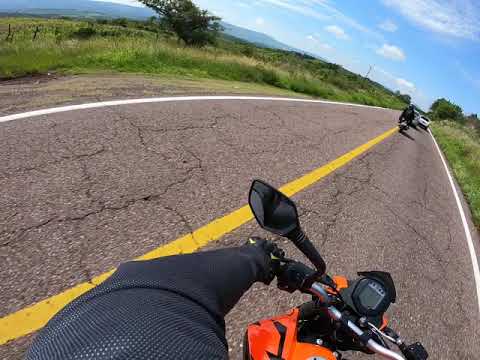The photograph captures a first-person perspective from a motorcyclist traveling on a two-lane asphalt highway with a solid yellow stripe running down its center. Taken with a fisheye lens, the image features curving white lines on the sides of the road that converge toward a curved horizon, producing a dramatic and immersive effect. In the foreground, the black handlebars with orange trim are visible along with the rider's sleeved left arm gripping the handlebar. The rider wears a black outfit, including a mesh long-sleeve shirt. The landscape on either side of the highway consists of grass, scrub, and a distant tree on the left side, complemented by a wooden fence with wiring. Ahead, another motorcyclist dressed in black is positioned directly on the yellow line, followed by two white cars in the distance. The sky above is a pale blue, streaked with delicate white clouds, adding to the expansive feel of the scene.